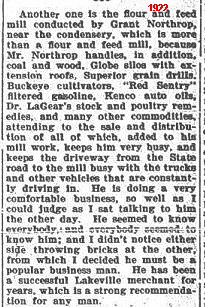The image depicts a small, rectangular clipping from an old newspaper, approximately two inches tall and one inch wide. The background is white with predominantly black text, complemented by a single piece of red text, '1922', situated in the upper right-hand corner, indicating the date. The content of the clipping details the operations of a flour and feed mill conducted by Grant Northrup near a condensary. This establishment is not limited to just milling; Mr. Northrup also manages coal and wood supplies, globe silos with extension roofs, superior grain drills, buckeye cultivators, red sentry filtered gasoline, Kenco auto oils, and Dr. Laguerre's stock and poultry remedies, among various other commodities. His extensive business involves significant milling work, requiring a busy driveway from the slate road to the mill with a constant flow of trucks and vehicles. Described as a successful and popular businessman in Lakeville, Northrup's operations keep him very occupied, suggesting a thriving and well-regarded enterprise.